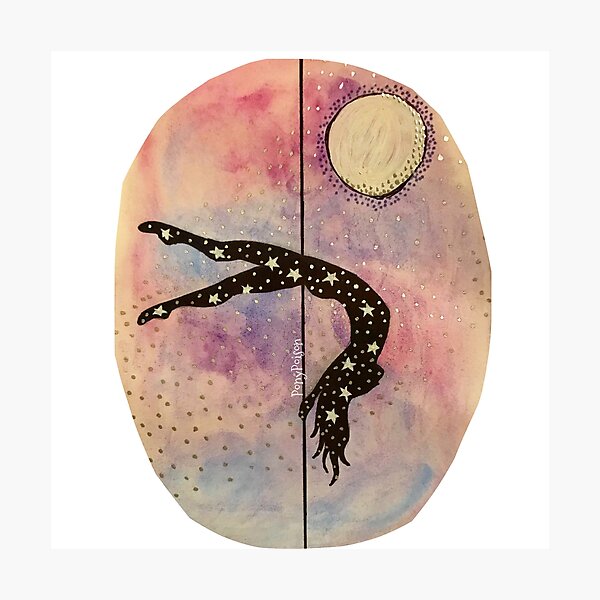This artwork is an abstract mixed-media painting that features a captivating pole dancer at its center. The silhouette of the pole dancer, rendered in black, is suspended upside down with her hair cascading down and her body gracefully bent around a horizontal black pole that cuts the oval canvas in half. Her legs are spread apart, showcasing her mastery and the dynamic nature of pole dancing. Intricately detailed inside her silhouette are numerous golden stars and dots, creating a starry, ethereal effect.

The composition is dominated by a large oval that sits in the center of a larger white square. This square is framed by a faint gray or tan border, providing a subtle but elegant boundary to the piece. In the upper right corner of the oval rests a sun-like figure, painted in an off-yellow hue with black dots encircling it, suggesting a radiant glow.

The background is an exquisite blend of watercolors with whimsical smudges of pink, purple, blue, and peach, interspersed with brown and golden dots that add texture and depth to the scene. This dreamy, pastel backdrop perfectly complements the striking silhouette of the dancer.

Apart from the visual elements, a mysterious inscription written close to the pole and the dancer in white letters could either indicate the artist's signature or a title. The piece is a celebration of movement, light, and contrast, drawing the viewer into its enchanting, otherworldly realm.